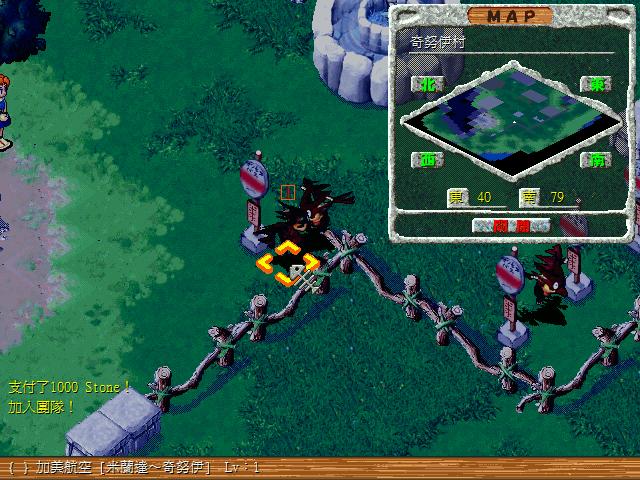This image is a screenshot of a video game with a prominently green landscape, suggesting a grassy map. The focal point includes a diagonal wooden fence resembling trees, stretching from the bottom and zigzagging towards the right. In the middle of the image, there is a noticeable gray round fountain, adding a significant landmark to the scene. Toward the top-right corner, a square mini-map labeled "map" is displayed, showcasing a diamond-shaped terrain. A yellow and orange cube-shaped cursor can be observed near the middle of the screen. Additional intriguing details include rocks scattered across the map, a fish skeleton draped over the fence, and various round signs positioned near the fence. Emblems and other icons are arranged above and below the mini-map, contributing to a rich and detailed interface.